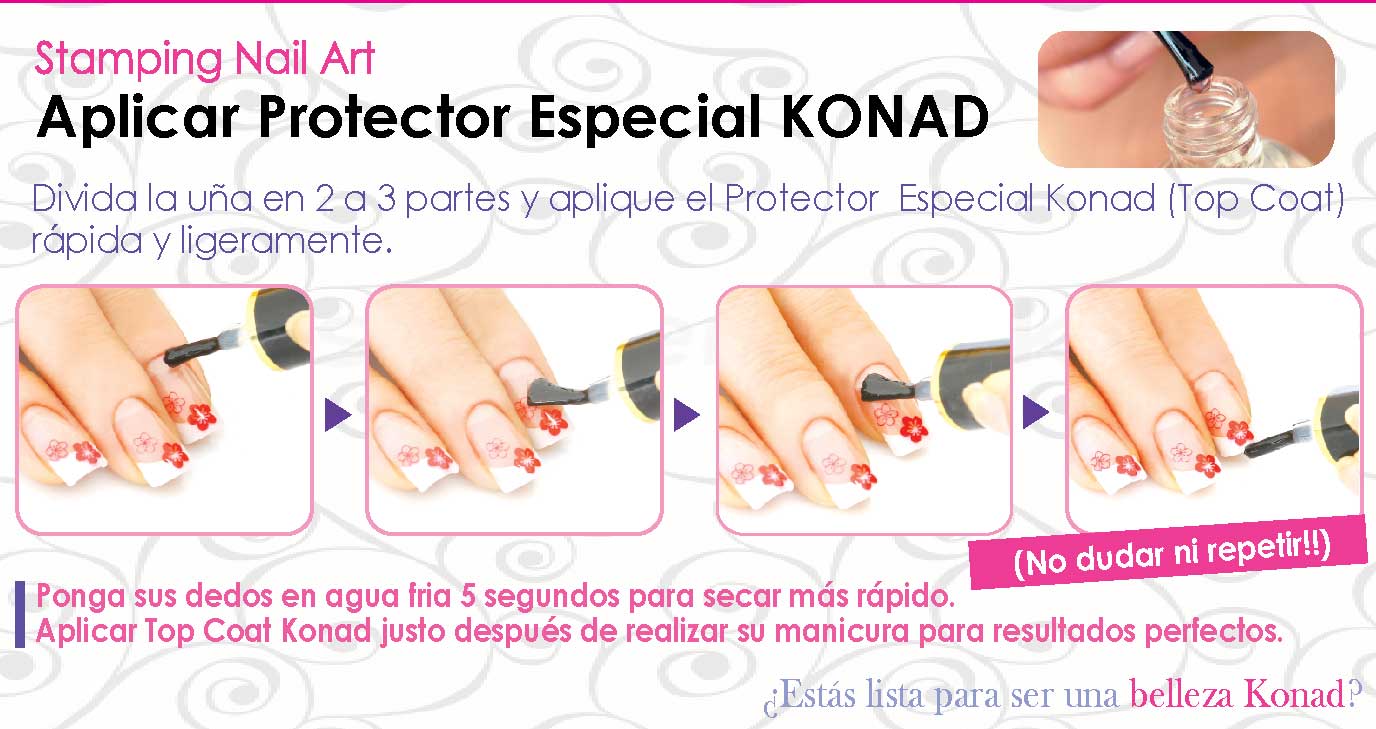This advertisement showcases a step-by-step guide for applying stamping nail art with a floral design. The top of the image features a thin horizontal purple line with the header "Stamping Nail Art" in purple, left-aligned text. Directly beneath, in black and also left-aligned, it states "Aplicar Protectar Especial Conad" with "CONAD" in all caps. On the right side, there's a small, rounded rectangular cutout depicting a person's finger lifting an applicator brush from a bottle. Below this, the Spanish text instructs to divide the nail into three parts and apply the special Conad top coat quickly and lightly. There are four sequential images displaying the stages of application, with a person's nails bearing white tips and a red floral pattern. These images each display the brush's position during the process. Additionally, swirling designs subtly decorate the background. The bottom of the image, in purple text, advises dipping fingers in cold water for 5 seconds to dry quicker and to apply the Conad top coat immediately after the manicure for perfect results.